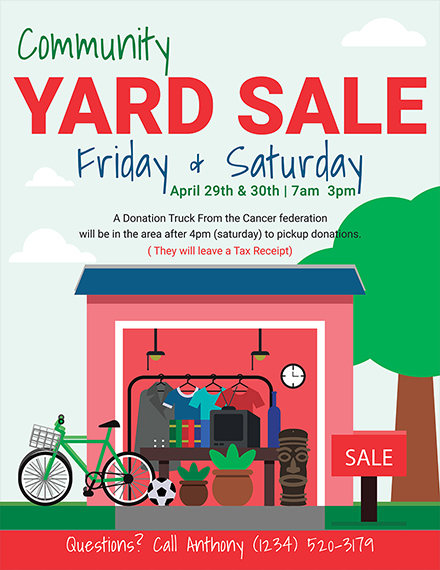The poster is a bright, cartoonish advertisement for a community yard sale happening on Friday and Saturday, April 29th and 30th, from 7 a.m. to 3 p.m. The words "Community Yard Sale" are prominently displayed at the top, with "Community" in green, "Yard Sale" in red, and "Friday and Saturday" in blue. Below the dates, in green text, it states the timing, and in black text, it mentions that a donation truck from the Cancer Federation will be available after 4 p.m. on Saturday to pick up donations. It also notes that tax receipts will be provided for donations. 

The central image features a small, pinkish shed or garage with a blue roof, showing various items arranged for sale inside and outside. Items depicted include a green and black bicycle, a rack of clothes, a small statue, a soccer ball, potted plants, a TV, books, and a gray table. On either side of the shed, there is green grass and a little walkway in the middle. To the right of the shed, there is a tree and a "For Sale" sign with red text on a black post. At the bottom of the poster, in red text, it says, "Questions? Call Anthony," followed by a phone number in white. The sky in the background is blue with some clouds, adding to the cheerful, inviting atmosphere.